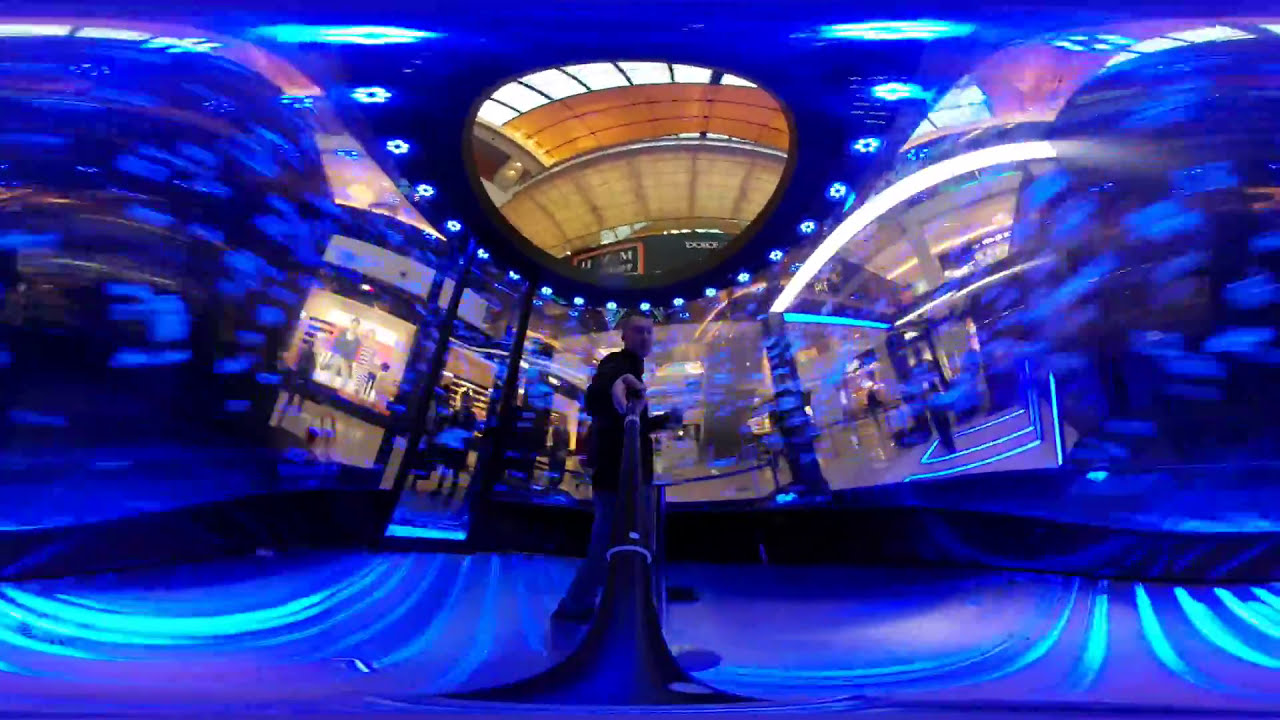In this panoramic, fisheye-lens image, a man with fair skin and short hair is featured walking through a shopping mall, holding a smartphone mounted on a selfie stick. The mall's interior is bathed in swirling blue lights that give both the floors and surroundings a dreamy, distorted quality. The man, dressed in a black shirt and lighter-colored jeans, appears slightly off-center in the photo, with a doorway entrance of a glass-fronted retail store visible to his left. Above him is a circular opening, possibly showing the roof of the mall or another part of the interior space. The vivid blue tones and the fisheye distortion give the entire scene an almost surreal appearance, accentuating the mall's spacious atrium-style roof and bustling shop fronts.